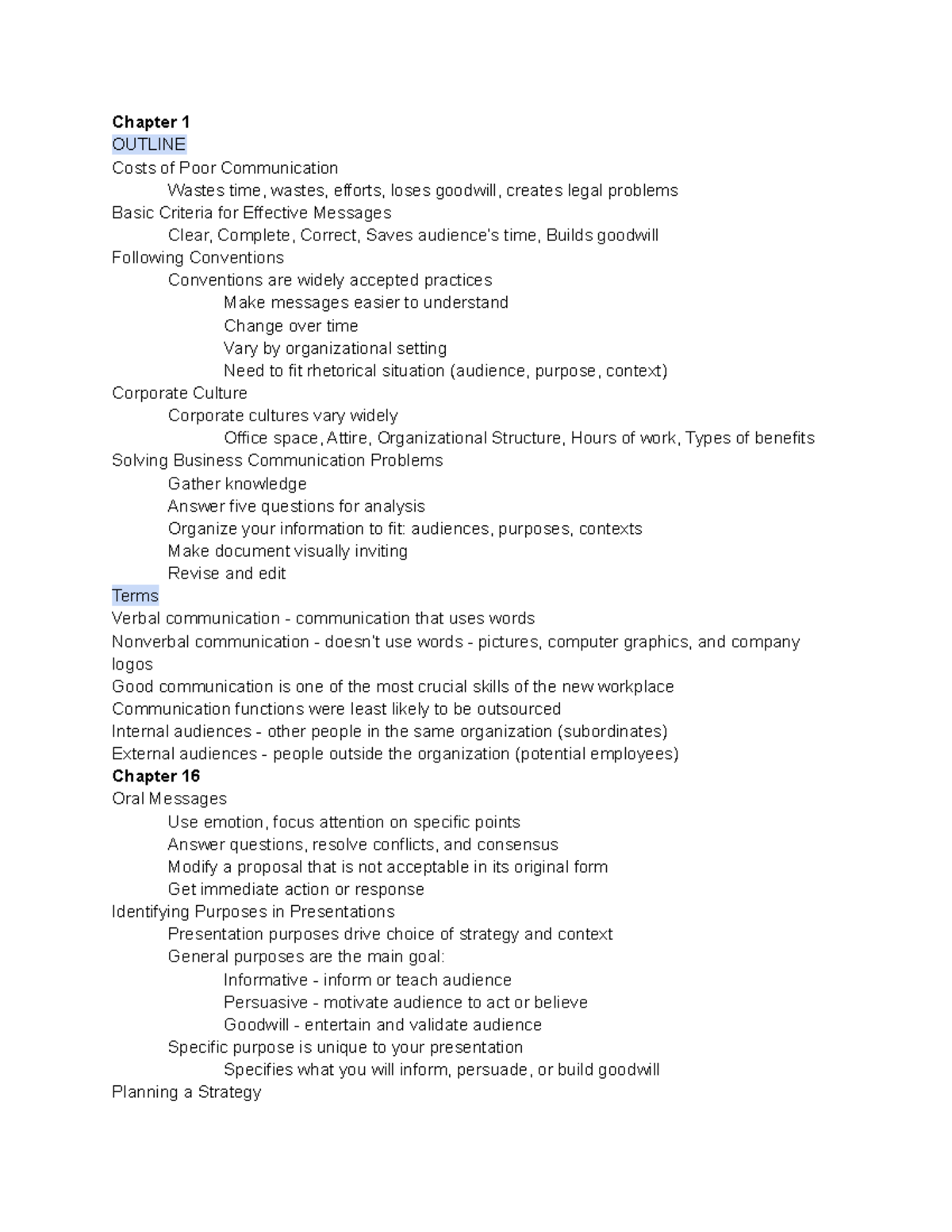### Detailed Image Caption:

The image features a clean, minimalist document outline on an entirely white background with black text. The layout is organized and features titles and sections clearly highlighted in blue.

**Title and Sections:**
1. **Chapter 1**: At the very top, the title "Chapter 1" is present, followed closely by the subtitle "OUTLINE," which is prominently highlighted in blue.

2. **Main Points and Subpoints:**
    - **Cost of Poor Communication**: This section outlines several detrimental effects, including:
        - Wasting time
        - Wasting effort
        - Losing goodwill
        - Creating legal problems

    - **Basic Criteria for Effective Messages**: This section lists essential characteristics of effective communication, such as:
        - Being clear
        - Being complete
        - Being correct
        - Saving the audience's time
        - Building goodwill

    - **Following Conventions**: This section explains the importance of conventions in communication:
        - They are widely accepted practices
        - Make messages easier to understand
        - Change over time
        - Vary by organizational setting
        - Need to fit the rhetorical situation (audience, purpose, context)

    - **Corporate Culture**: This section highlights diverse aspects of corporate culture:
        - Office space
        - Attire
        - Organizational structure
        - Hours of work
        - Types of benefit

    - **Solving Business Communication Problems**: This critical section provides a structured approach to addressing business communication issues:
        - Gather knowledge
        - Answer five analysis questions
        - Organize information to fit the audience, purpose, and context
        - Make the document visually inviting
        - Revise and edit

3. **Terms**: Highlighted in blue, it introduces definitions and important concepts:
    - **Verbal Communication**: Communication using words
    - **Nonverbal Communication**: Communication without words, including pictures, computer graphics, and company logos
    - **Importance of Good Communication**: Emphasizes that good communication is a crucial skill in the modern workplace and is least likely to be outsourced
    - **Internal Audiences**: Defines as other people within the same organization (e.g., subordinates)
    - **External Audiences**: Defines as people outside the organization (e.g., potential employees)

4. **Chapter 16: Oral Messages**: This section is dedicated to the nuances of delivering oral messages:
    - **Using Emotion**: To focus attention on specific points, answer questions, resolve conflicts, and build consensus
    - **Modifying Proposals**: For proposals that are not acceptable in their original form
    - **Getting Immediate Action or Response**

5. **Identifying Purposes in Presentations**: This part provides guidance on the purposes and strategies of presentations:
    - Presentation purposes drive the choice of strategy and context
    - General purposes include informing (teaching the audience), persuading (motivating the audience to act), and building goodwill (entertaining and validating the audience)
    - Specific purposes are unique to each presentation and specify what you will inform, persuade, or build goodwill about.

The entire outline is meticulously organized, lending to easy readability and clear comprehension of each section.